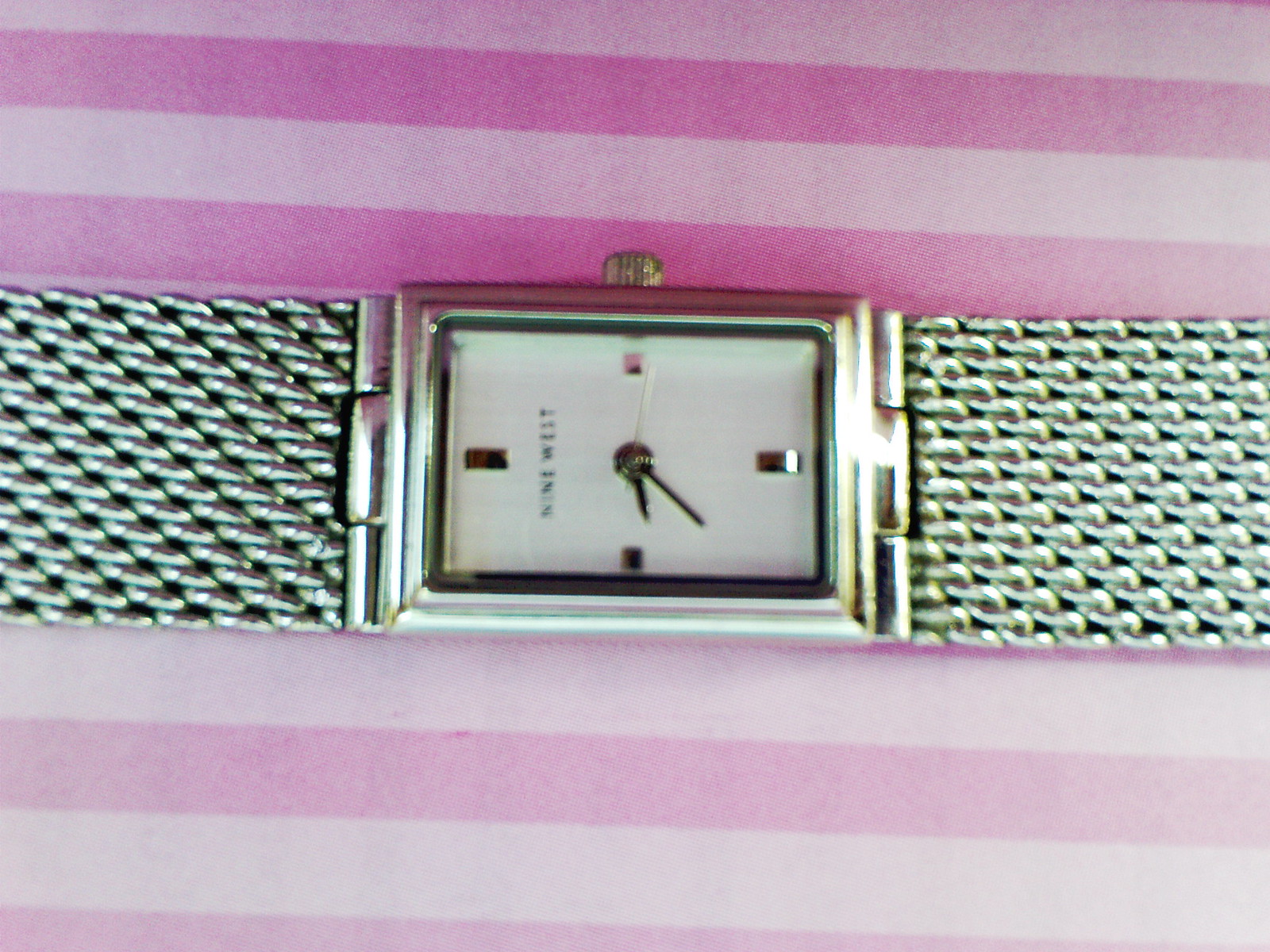This is a photograph of a wristwatch with a woven, braided metal band resembling a chain link, silver in color. The band extends flat across a pink striped background, with alternating light and dark pink stripes. The watch is centrally positioned and lies horizontally, showing the dial nearly square in shape and tilted slightly to depict a time around 8:40. The dial is white, adorned with silver lines at the 12, 3, 6, and 9 positions, lacking numerical markers. The brand name on the dial reads "Nine West" and is situated above the center of the watch face. The watch face and a portion of the band are visible in the middle of the image, with equal space above and below, emphasizing the watch as the focal point.